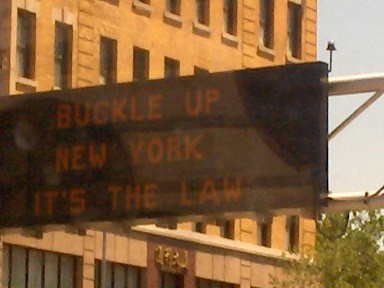This is a somewhat dated and blurry color photograph, likely taken from within a vehicle, depicting a black digital traffic sign that reads in red lettering, "Buckle up, New York. It's the law." The sign, supported by a post visible on the right side of the image, is a public safety announcement typically seen on highways or roads. In the background, there stands a very tall, old brownstone building with some type of indistinct gold lettering over an entryway. The upper stories of this building are prominently featured, although the exact height cannot be discerned. To the right of the building, the sky appears clear and light blue. At the bottom of the photograph, a portion of trees is visible. Additionally, a small pole-mounted sensor, possibly a traffic camera or speeding sensor, can be seen in the image. There are no people, animals, birds, vehicles, or bodies of water present in this photograph.